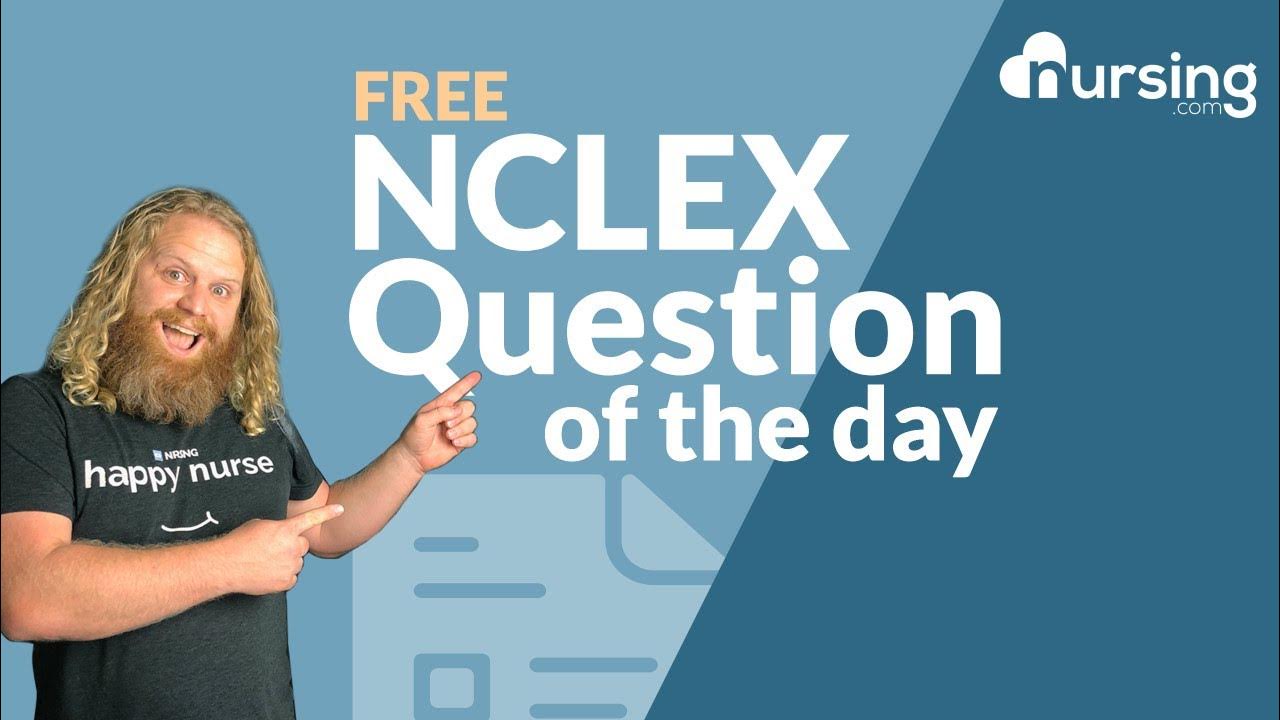The image is a digital slide, resembling a presentation from Google Slides or Microsoft PowerPoint. The slide features a black background bordered in blue, with a dark blue panel as its frame. At the top, "Question of the Day" is prominently displayed in large white text. Below, a detailed nursing scenario is presented: "A nurse is preparing to irrigate a patient's nasogastric (NG) tube. She has assessed the patient's abdomen and confirmed the tube's tip is in the stomach. After drawing 30 milliliters of normal saline into a syringe, the nurse prepares for the next step." This is followed by a multiple-choice question asking which action the nurse should take next. The options are: 
A) Attach the syringe to the NG pigtail and administer 30 milliliters of normal saline.
B) Assess for kinks or other signs of occlusion in the tubing.
C) Ask the patient to open her mouth and swallow.
D) Clamp the suction and disconnect the tube.
The slide is signed "NRSNG" in white text at the bottom right corner.